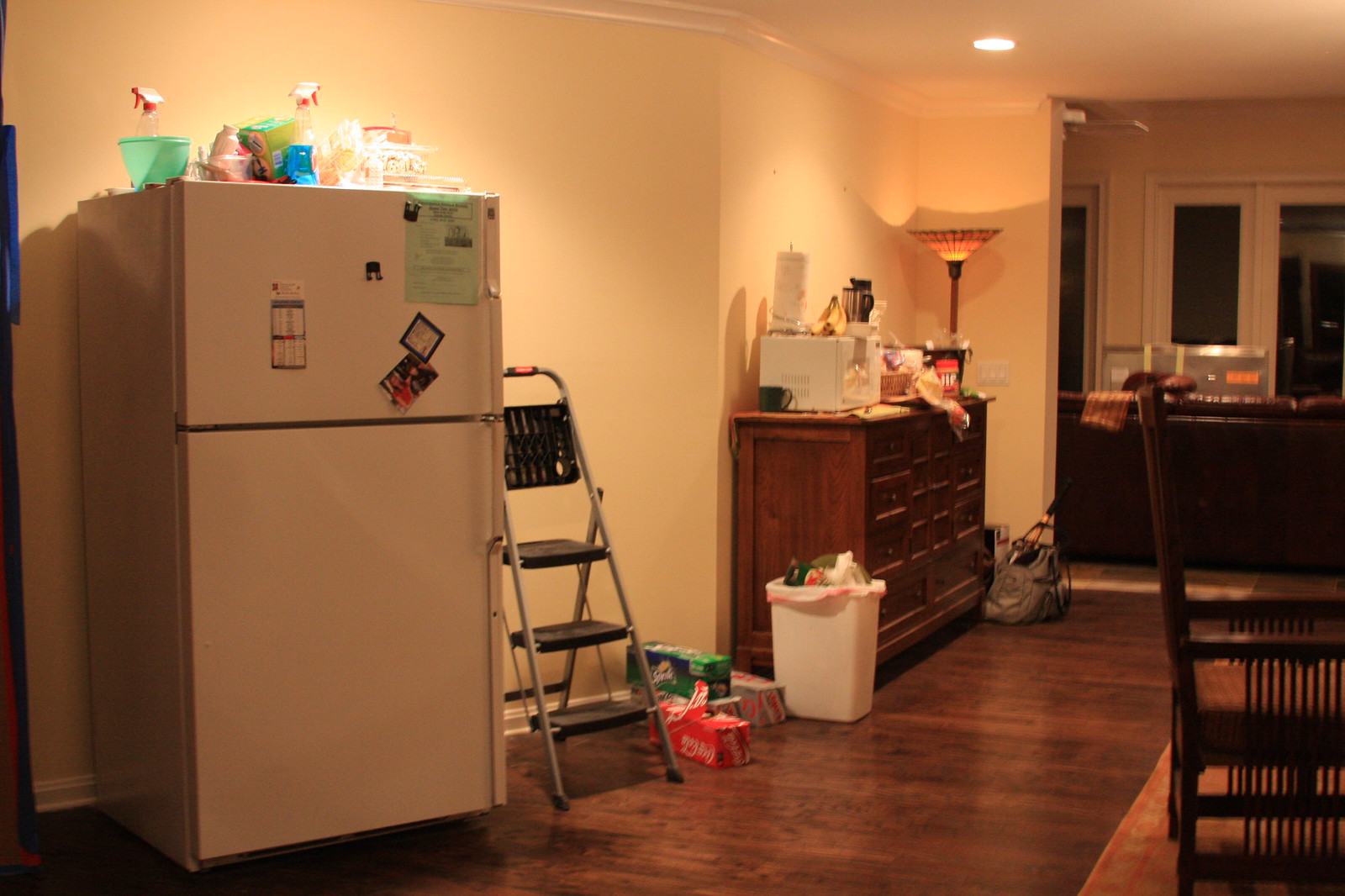In the image, a cozy corner of a home is depicted. Dominating the left side is a white refrigerator positioned against a tan-colored wall. The room is dimly lit, with strategically placed lamps providing a warm, ambient glow. The top of the refrigerator is cluttered with various items, while its front surface is adorned with several magnets. To the right of the refrigerator, a three-tier step stool is propped open against its side.

On the floor, multiple boxes of soda pop are visible: an orange box, a green one, and another with an orangish hue. Nearby, a white trash can with a pink-lined white trash bag is filled to the brim with discarded items. 

Adjacent to the refrigerator and step stool, a wooden chest of drawers stands against the wall, its surface also laden with assorted belongings. The floor is covered in dark brown hardwood, adding to the room's warm and inviting atmosphere. A hardwood chair is also visible, complementing the overall aesthetic. This detailed depiction captures a lived-in, functional space with a touch of everyday clutter.